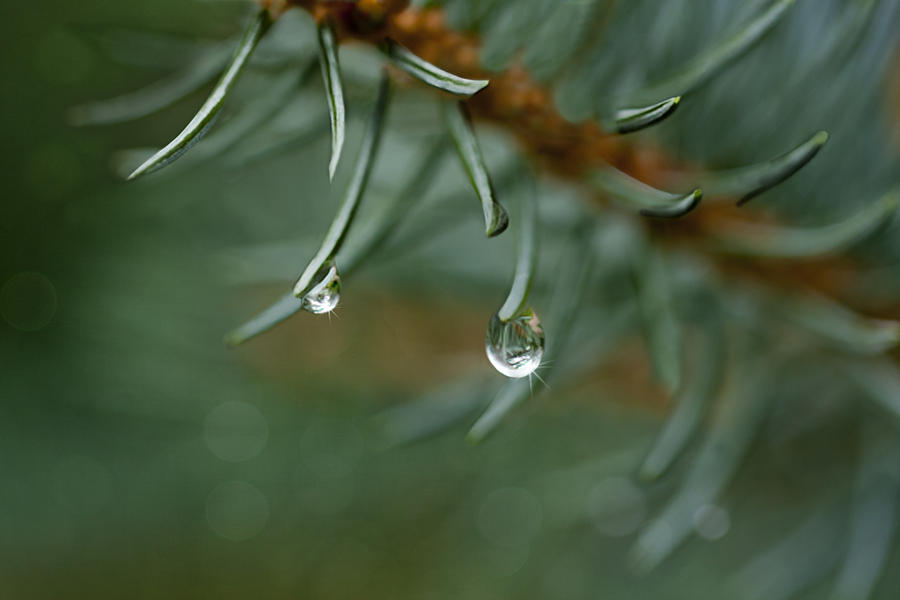This image is an extremely up-close, detailed photograph of a pine tree branch with two sparkling water droplets hanging precariously from the tips of dark green pine needles. The brown stem extends diagonally from the top left to the center right, anchoring the needles that fan out delicately. The background is a blur of varying shades of green and brown, enhancing the sharp focus on the foreground. Only the very tips of the pine needles and the water droplets are in clear focus, capturing the luminous droplets that glisten like diamonds. One droplet, slightly larger and more teardrop-shaped, dangles closer to falling, while the other clings more tenaciously to its needle. The overall play of light on the droplets and needles creates a shimmering effect that stands out against the soft, dreamy backdrop.